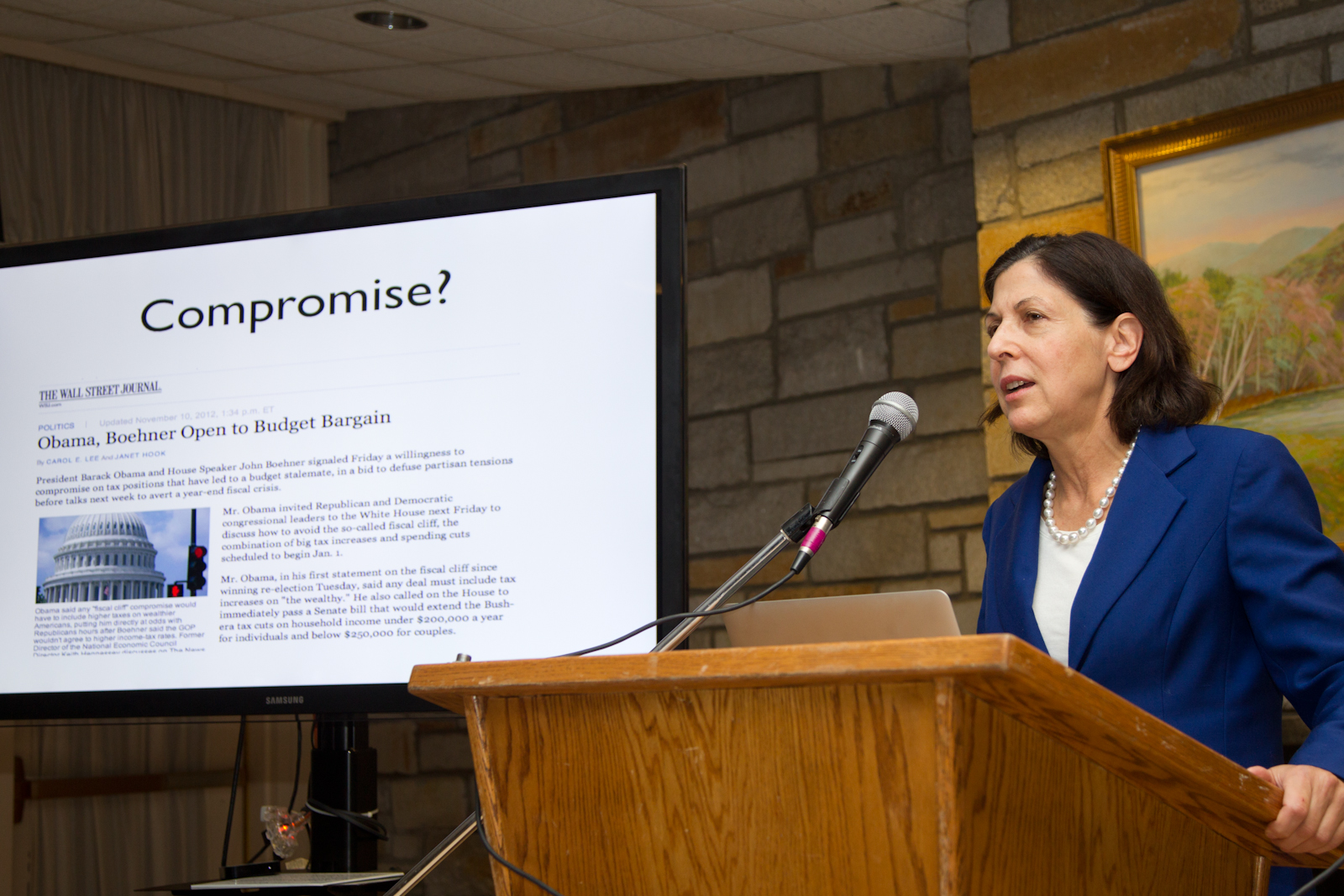In this image, a woman in her late 20s stands at a wooden podium equipped with a microphone. She is dressed in a white shirt beneath a blue blazer, which is buttoned at the bottom, and accessorized with a pearl necklace. Her dark brown, shoulder-length hair frames her face as she grips the podium with her left hand. Behind her, a tan and rust-colored brick wall features a gold-framed painting depicting an autumn landscape with a forest and a lake, where the leaves exhibit shades of pink, yellow, and green. To her right, a flat-screen TV with a black trim displays a news article from the Wall Street Journal, with a white background and the word "compromise?" in bold black text at the top. Specifically, the article headline reads "Obama-Boehmer open to budget bargain." Although the crowd is not visible, it appears she is addressing a small audience.